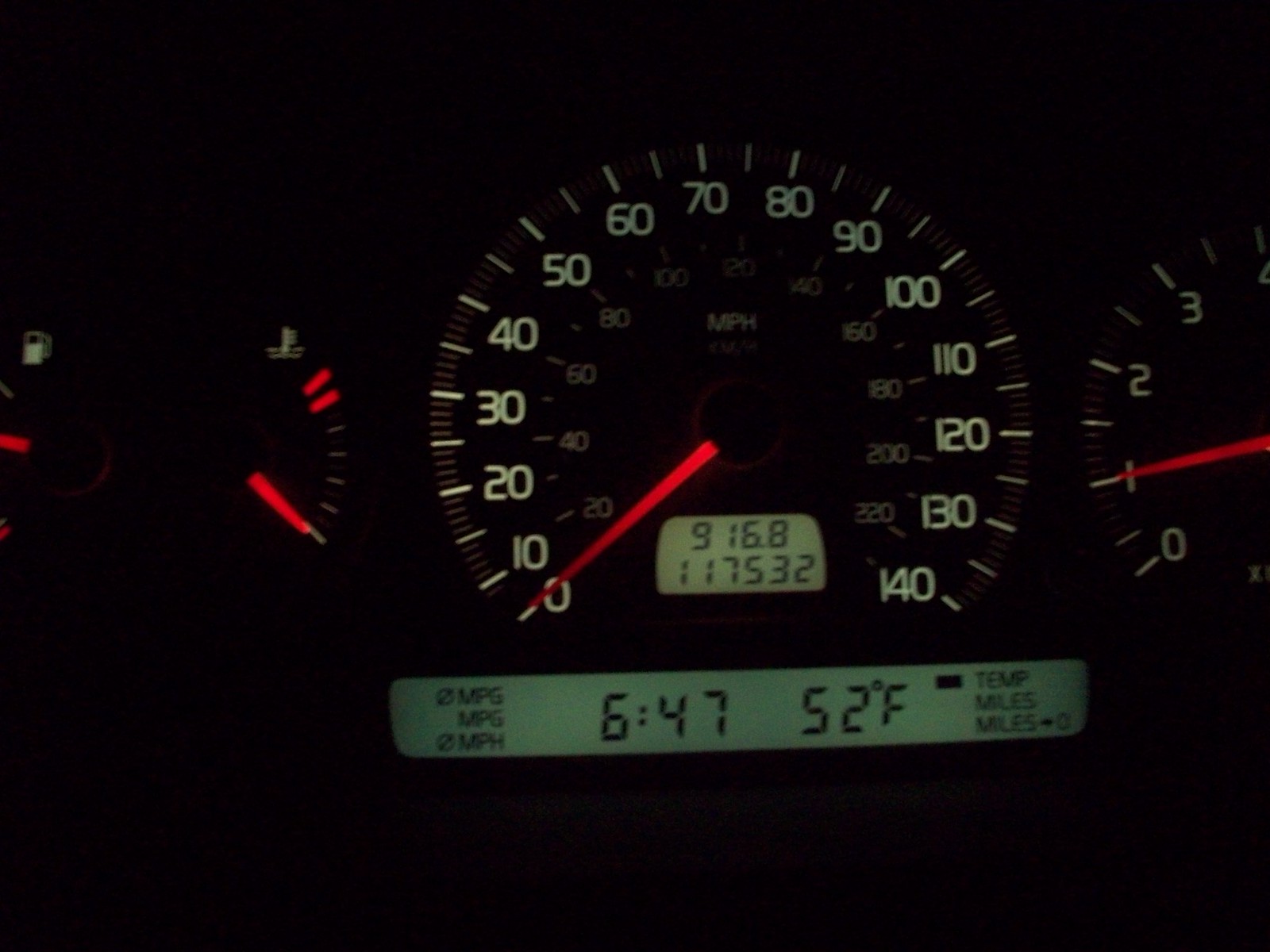This photo, taken at night inside a vehicle, focuses on the illuminated instrument cluster, featuring the speedometer prominently centered. The speedometer needle rests at zero miles per hour, indicating the vehicle is stationary. Two digital displays are integrated within the speedometer. The top display, adjacent to the red needle, shows the trip distance of 916.8 miles, while directly below, the odometer reads 117,532 miles, reflecting the total mileage of the vehicle. Below these readings, a secondary digital screen displays the current time, 6:47, and the external temperature, 52 degrees Fahrenheit, along with a bar indicating that this temperature is the current setting. To the left side of this display, text reads 'mile', 'MPG', and 'MPH', though it is currently set to MPG and MPH. Additionally, part of the tachometer is visible to the right, showing the engine idling at 1,000 RPMs, with markings extending up to 4,000 RPMs. Left of the speedometer, a lit icon of a gasoline pump and a temperature gauge are also partially visible, adding to the detailed snapshot of the vehicle's dashboard.